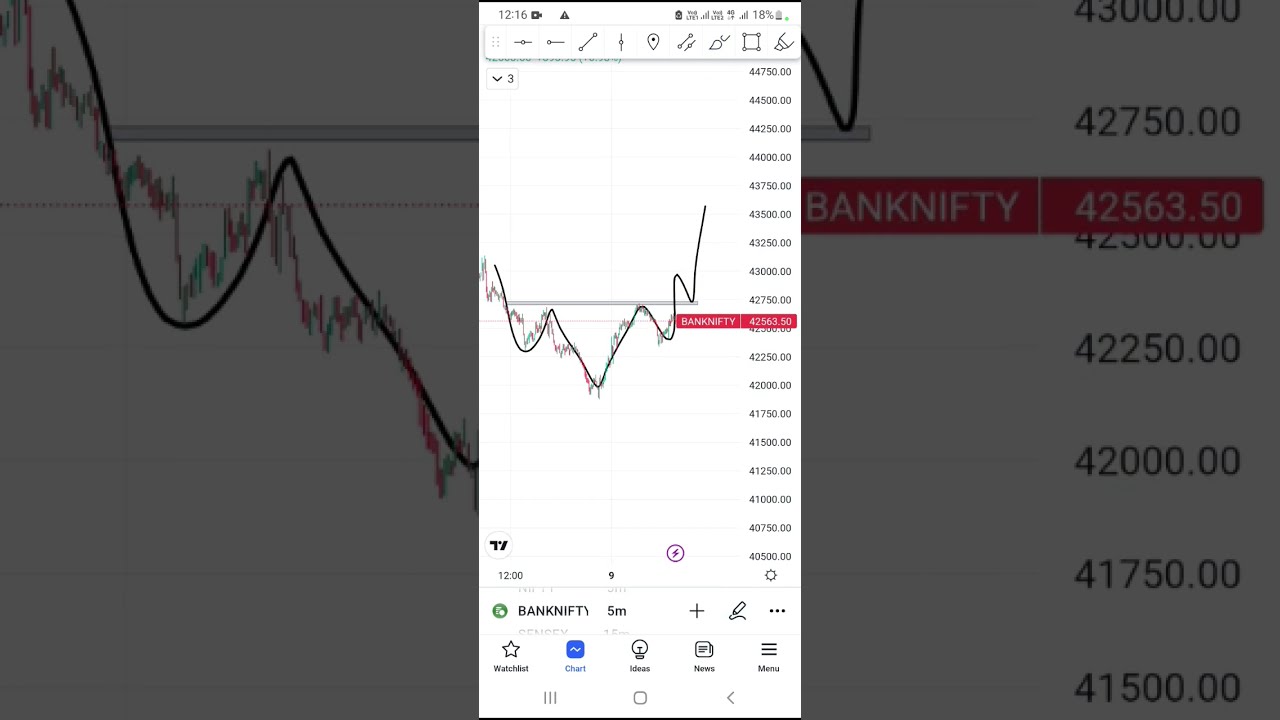The image is a vertical screenshot from a cell phone displaying a financial graph of a company called Bank Nifty. Centered prominently, the graph’s background is bright and legible, while the surrounding areas are darker and shaded. The graph itself is a black line chart that fluctuates between 44,750 at the top and 40,500 at the bottom, with specific points such as dipping to 42,000 and peaking at about 43,700. This line graph shows multiple spikes and dips, akin to heartbeat signals, and is set against faint lateral lines marking the numerical values on the right side. At the top of the phone screen, there are standard icons indicating battery life (18%), WiFi, and other status symbols. The bottom section of the graph displays various icons and options such as a star for a watch list, a blue box labeled chart, a light bulb for ideas, a news section, and the typical three horizontal bars for a menu. Additionally, cursor-editing buttons like highlight and paint are visible near the top edge. The left-hand side of the screen also features a back button, alongside symbols and editing tools. Overall, the screenshot encapsulates a detailed view of Bank Nifty's financial data visualized through a line graph on a mobile device interface.